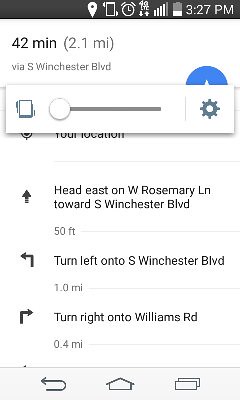This detailed screenshot from an Android phone captures a navigation screen from an app like Google Maps, detailing a route with specific turn-by-turn instructions. At the top of the screen, there's a black bar showing various status icons: a white teardrop symbol indicating GPS is active, a phone icon suggesting vibration mode with surrounding lines, an alarm clock icon for a set timer, "4G LTE" with accompanying up and down arrows for mobile data, full four bars of signal strength, and a battery icon indicating approximately 25-33% battery remaining. The time reads 3:27 p.m.

Beneath this status bar, a navigation instruction states "42 minutes (2.1 miles) via South Winchester Boulevard." Below, there’s a settings bar with a cogwheel and a slider, likely for adjusting vibration settings, and a symbol indicating vibration mode again.

The directions detailed on the white background with black text instruct:
1. Head east on W Rosemary Lane toward South Winchester Boulevard for 50 feet.
2. Turn left onto South Winchester Boulevard for 1.0 mile.
3. Turn right onto Williams Road for 0.4 miles.

At the bottom of the screen are navigation buttons for the phone: a curved left arrow for back, a house icon for home, and an overlapping squares icon for recent apps.